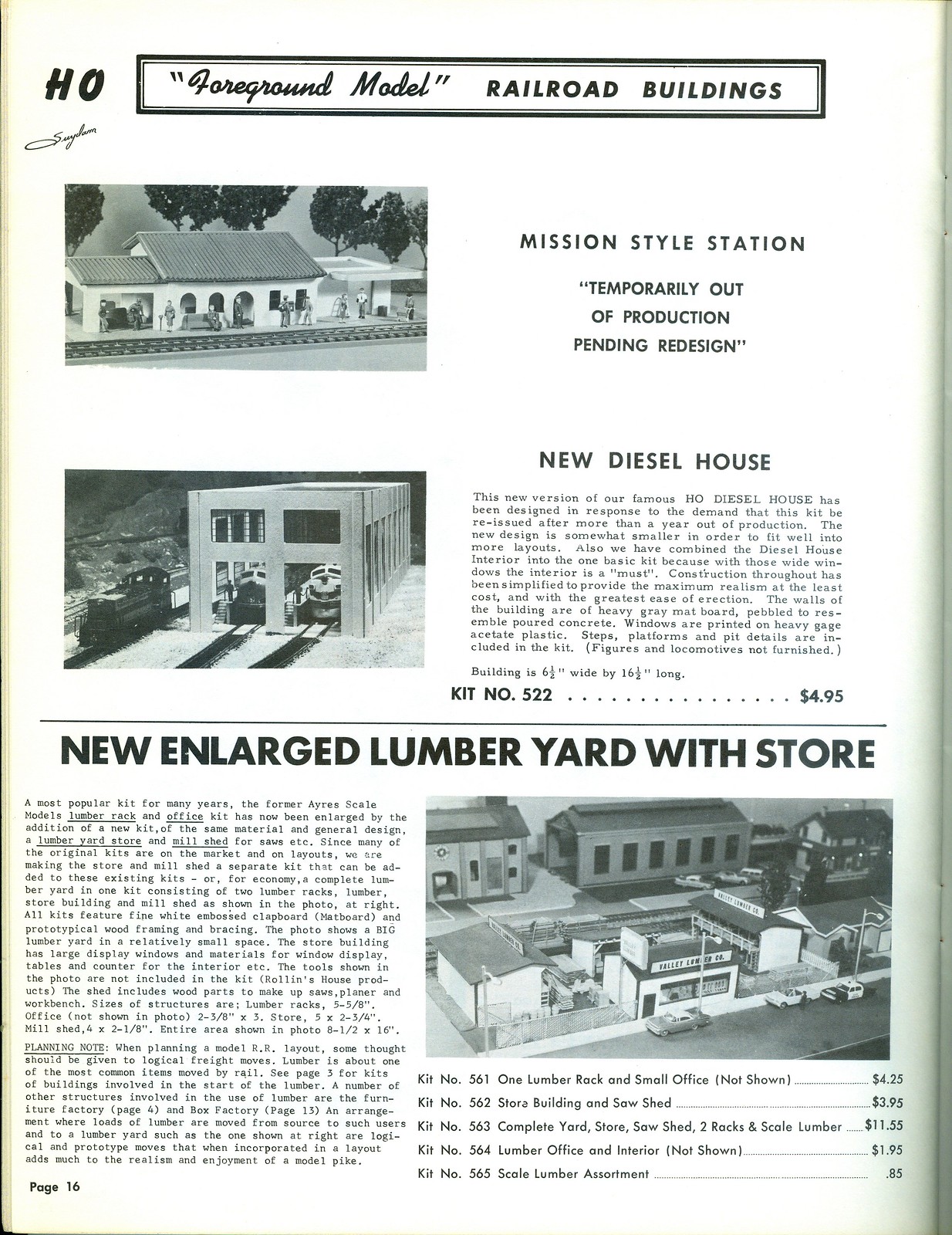This black and white image captures a page from an old catalog or booklet, specifically page 16. The top of the page is headlined with the title "Foreground Model Railroad Buildings." The page features photographs and descriptions of various model railroad building kits.

At the top, a photograph showcases a Mission-style station with a note stating that it is temporarily out of production pending a redesign. Below this, there is a photograph of a long, rectangular building labeled "New Diesel House." The description highlights that this updated version of the renowned diesel house kit was reintroduced due to high demand after being out of production for over a year. The new design is slightly smaller, making it more compatible with a wider range of model train layouts. This New Diesel House kit is priced at $4.95.

Further down, the catalog features a "New Enlarged Lumberyard with Store." Details about the prices are noted: the diesel house kit costs $4.95, the lumber back and small office are priced at $4.25, and the complete lumberyard, which includes a store, saw shed, two stacks, and scale lumber, is available for $11.55.

The exact publication year of the catalog remains unspecified. The page provides a glimpse into the variety of building kits available for model train enthusiasts and their associated costs, emphasizing the detailed craftsmanship and historical context of these miniature structures.